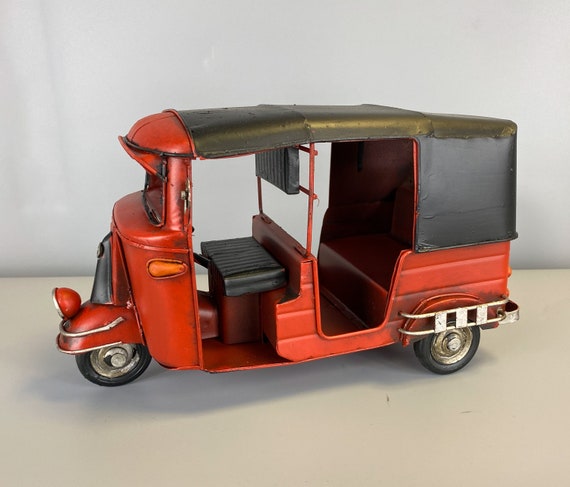The image showcases a detailed toy representation of a red three-wheeled tuk-tuk. The front section of the vehicle features silver decorative bars surrounding the mudguard and silver centers on both the front wheel and visible rear wheels. A prominent red headlamp adorns the front, adding to the toy’s realistic appearance. The cab, visible through the windscreen, includes a black seat and various controls, giving an authentic touch to the driver’s area. A divider separates the driver’s area from the passenger section, which has a supportive headrest for the driver. Behind the driver, there is a spacious back seat designed to accommodate two passengers. Notably, a ladder-like structure extends over the rear wheel, serving as a protective barrier to prevent objects from interfering with the wheel. The entire vehicle is topped with a sleek black roof, covering both the driver and passenger areas.